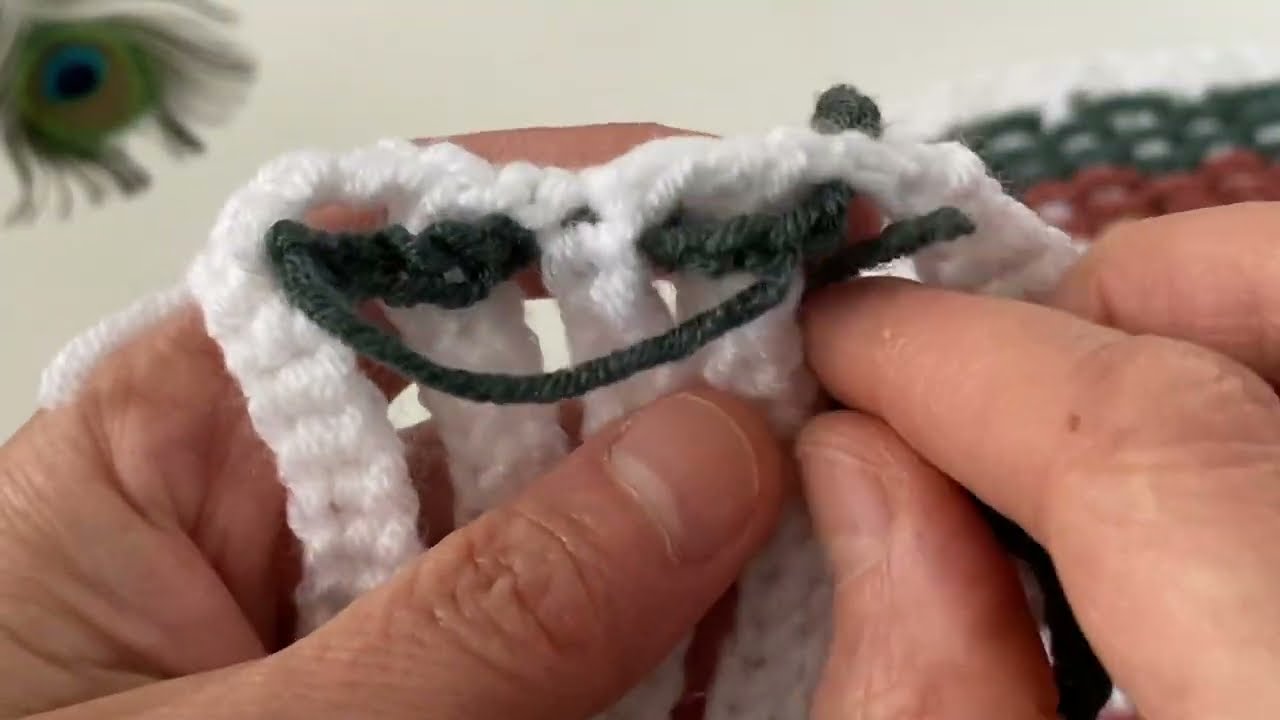This image features a close-up of two hands with pale, chapped skin and recently cut nails, suggesting the person might be Caucasian. The hands are engaged in a crocheting project, as indicated by the lack of visible knitting needles. They are weaving together strips of white and dark green yarn, with five white crocheted segments arranged in a row. Dark green thread is intricately braided through the middle three white strips, connecting them. In the background on the left side, there is a blurry, peacock-colored object, possibly a dreamcatcher, and a cream-colored wall. In the upper right corner, a glimpse of the finished blanket can be seen, composed of sections of white, dark green, and darker red yarn. The meticulous detail in the crocheting suggests the creation of a blanket.